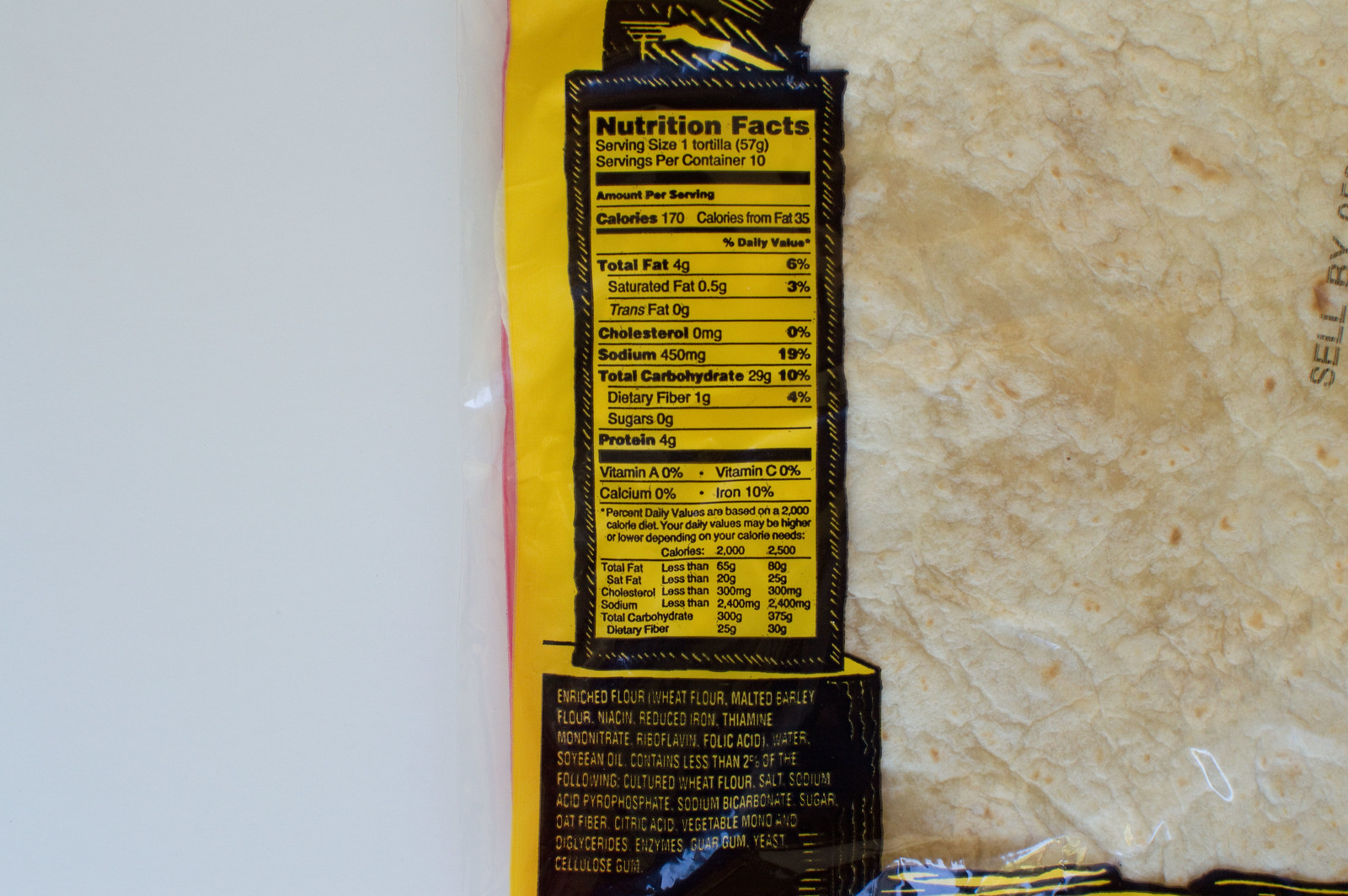The image features a partial view of a tortilla package, focusing on the nutrition label. The label is presented on the side of the package, with the colors black and yellow prominently displayed. The tortilla itself is visible through a transparent section of the packaging. The package rests on a white surface, likely a countertop. The nutrition facts indicate that a serving size of one tortilla contains 170 calories, with 35 calories coming from fat. It lists 4 grams of total fat, including 0.5 grams of saturated fat and no trans fat. Cholesterol content is zero, while sodium is registered at 450 milligrams. The tortilla includes 29 grams of carbohydrates, 1 gram of dietary fiber, and no sugars. It also provides 4 grams of protein. The ingredients list is located at the bottom of the label.